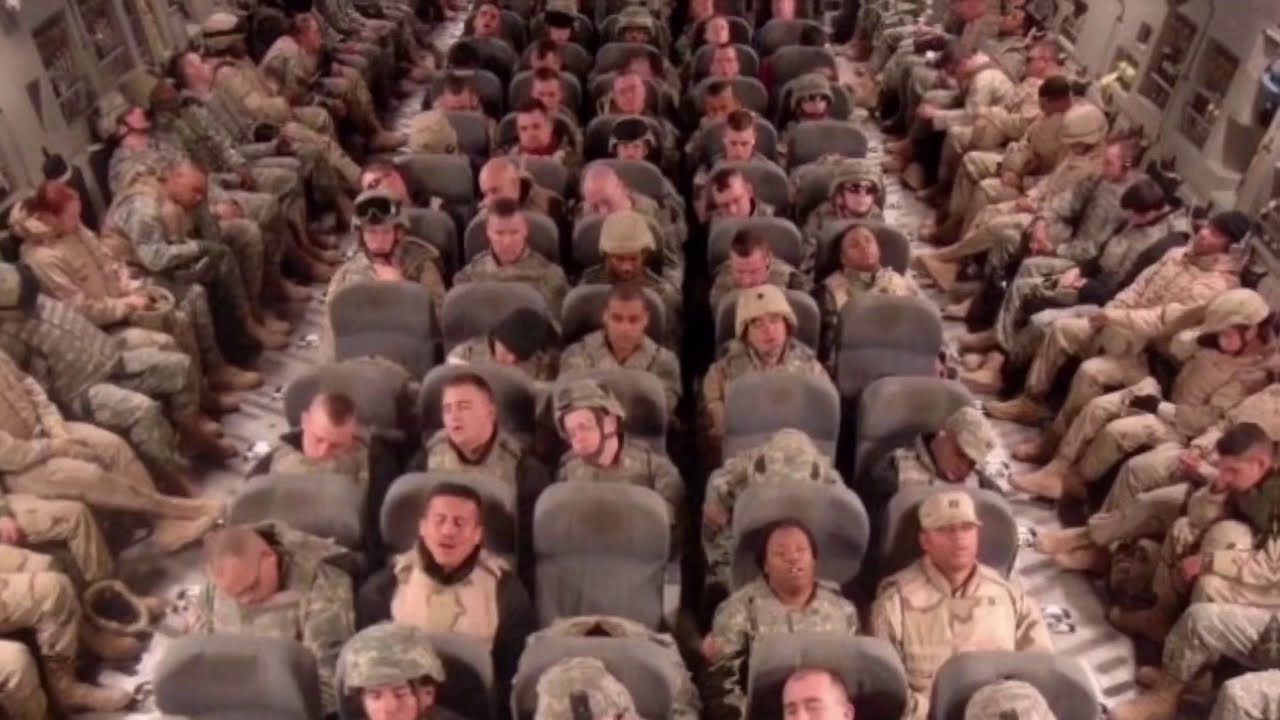This detailed overhead photograph captures the interior of a large military transport aircraft. In the center, you see rows of five seats each, extending back for at least 11 rows, all filled with military personnel in uniforms. Some individuals are resting with their heads back and eyes closed, while others are engaged in conversation, leaning towards their neighbors. The mixture of attire includes uniforms, helmets, and hats. Flanking these central rows, there are single rows of seats along both the right and left sides of the plane, where additional military personnel sit perpendicular to the main group, their backs against the aircraft's interior walls. The color palette is dominated by muted tones of gray, beige, brown, tan, white, and black, reflecting the utilitarian design of the military setting.